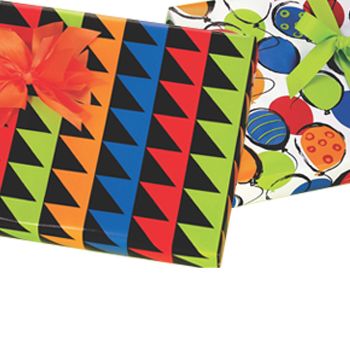This image features two distinctively wrapped presents set against a stark white background. The present on the left showcases a repeating pattern of black triangles arranged in rows, interspersed with vertical columns of light green, red, blue, and orange colors. It is neatly adorned with an orange bow at its center. The present on the right, partially overlapped by the first, is wrapped in paper with a white background decorated with colorful balloons. The balloons vary in design: some are blue with yellow stripes, others are orange with red dots, and there are solid blue and green balloons as well. Completing the festive look, this present features a lime green bow positioned at the upper right-hand corner.